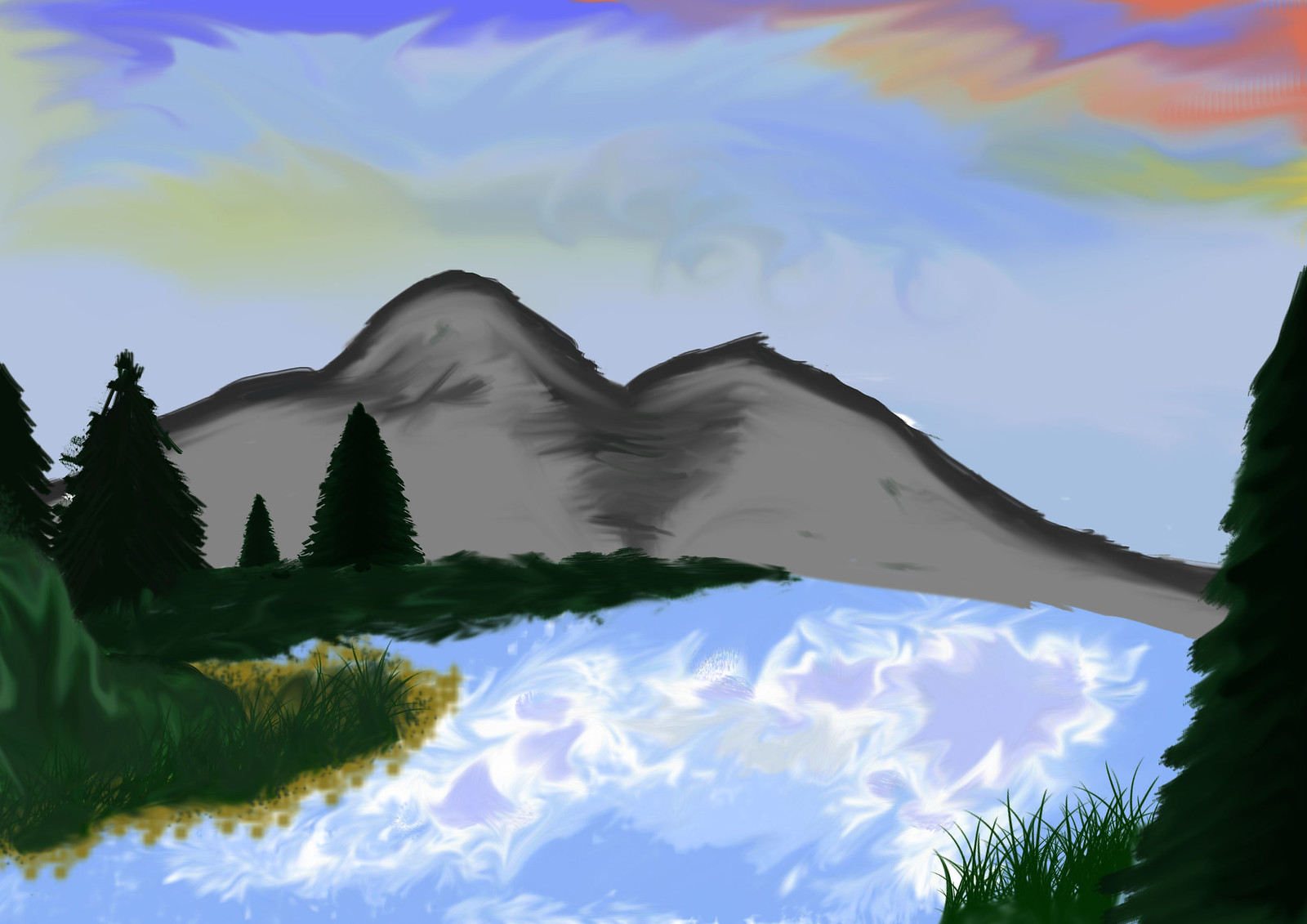This captivating artwork, possibly created through traditional painting methods or digital software, presents a mesmerizing landscape that blends lifelike elements with more surreal touches. Dominating the background is a gray mountain, its rugged silhouette sharply outlined in black, standing majestically in the distance. The heart of the scene features a serene blue stream, with hints of purple, giving the impression of a sky's reflection on the tranquil water.

In the bottom right corner, vibrant green grass and a solitary pine tree anchor the composition, adding depth and realism. On the left side of the painting, additional pine trees, shadowy and distant, populate another grassy patch, enhancing the sense of a sprawling valley.

The sky above is a breathtaking mosaic of colors, evoking the beauty of a sunset. It transitions through various shades of blue, intermingled with strokes of yellow, indigo, purple, red, and pink, especially pronounced towards the upper right section of the canvas. This rich palette infuses the scene with a dreamlike quality, balancing between reality and imagination.